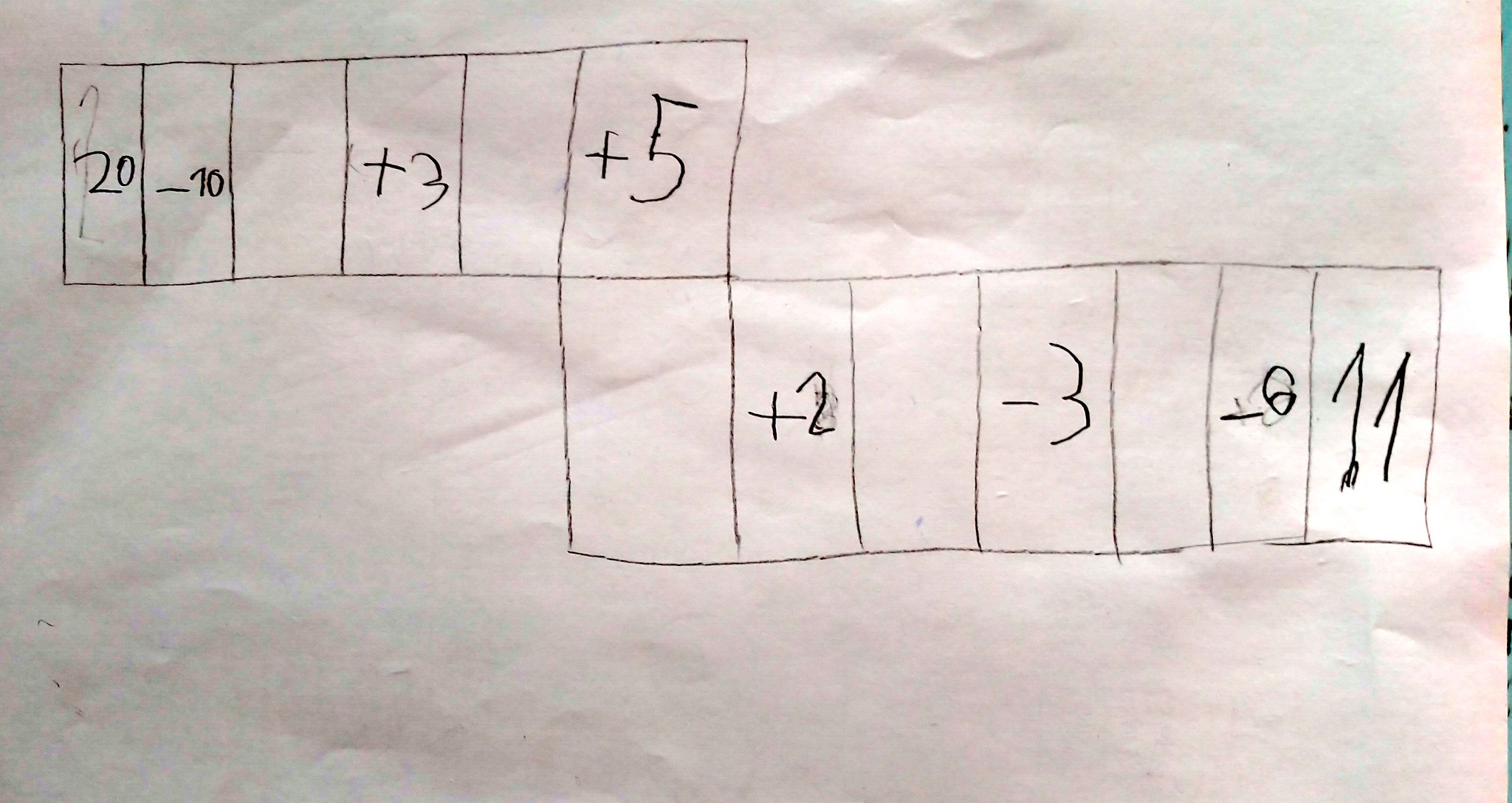The image depicts a hand-drawn grid of vertically-oriented rectangles, each outlined in pencil. Despite variations in shape, all rectangles maintain a generally vertical alignment, although some lines are not perfectly straight. The background is a plain white sheet of paper, illuminating any unmarked, empty rectangles with a white fill.

In the top-left corner of the image, six connected rectangles form a vertical column. The contents, in order from top to bottom, are as follows:
1. A rectangle with the number "20" written inside.
2. A rectangle with "-10" written inside.
3. An empty rectangle, revealing the white paper background.
4. A rectangle labeled "+3."
5. Another empty rectangle.
6. A rectangle marked "+5."

A seventh rectangle connects to the bottom of this column, leading to a horizontal sequence of six additional rectangles extending to the right. The details for this row, from left to right, are:
1. An empty rectangle.
2. A rectangle with "+2" inscribed.
3. An empty rectangle.
4. A rectangle marked "-3."
5. Another empty rectangle.
6. A rectangle labeled "-6."
7. Finally, a rectangle exhibiting the number "11" prominently written in large characters.

Overall, the composition features a thoughtful arrangement of numbers and symbols amidst intermittent empty spaces, all against a clean white background.